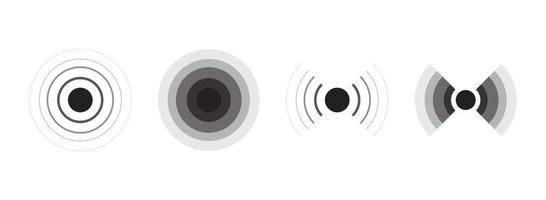The image features a sequence of four black and white geometric sketches lined up in a row against a white background. Each sketch prominently includes circular designs. 

The first sketch showcases a bullseye pattern with concentric rings that darken as they approach a solid black center. It starts with lighter outer rings that progressively become thicker and darker towards the middle.

The second sketch also resembles a bullseye but with a more varied grayscale progression. The center is dark, surrounded successively by dark gray, medium gray, and lighter gray rings.

The third sketch includes a central dark gray circle, flanked by semi-circular lines that resemble sound waves or rainbows radiating outward in half arcs on both sides. The lines are prominently outlined.

The fourth sketch mirrors the design of the third but with filled-in semi-circular sections that create a pattern of two grayscale rainbows on either side of the central dark gray circle, transitioning through light gray, dark gray, black, white, and back to black again.